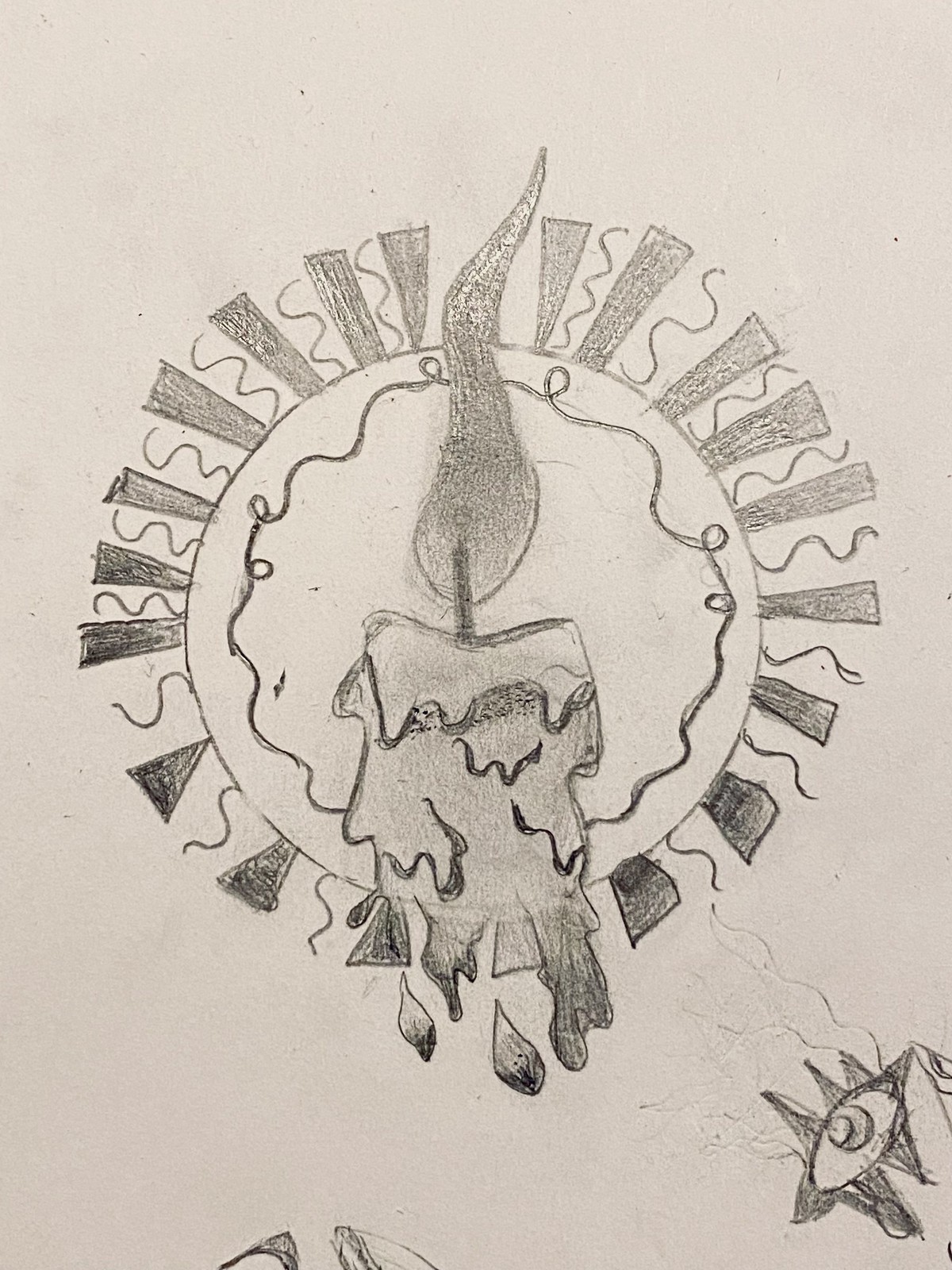This is a detailed pencil drawing on an off-white background, depicting a melting candle with a large flame that is exaggerated in size, extending above the wax holder. The wax appears to be dripping, forming teardrop shapes beneath the candle. The central composition of the drawing is set within an abstract decorative ring. This ring features a blend of geometric patterns, including straight lines, rectangles, and squiggly lines that create an intricate clock-like design. The center of this circular design itself also includes a squiggly-lined circle. In the bottom corner of the image, there lies a distinct human eye symbol, characterized by aggressive, triangular shapes for eyelashes that resemble teeth. The eye has three of these triangles on top and two on the bottom. Some markings appear partially erased, adding to the abstract, textured nature of the artwork.